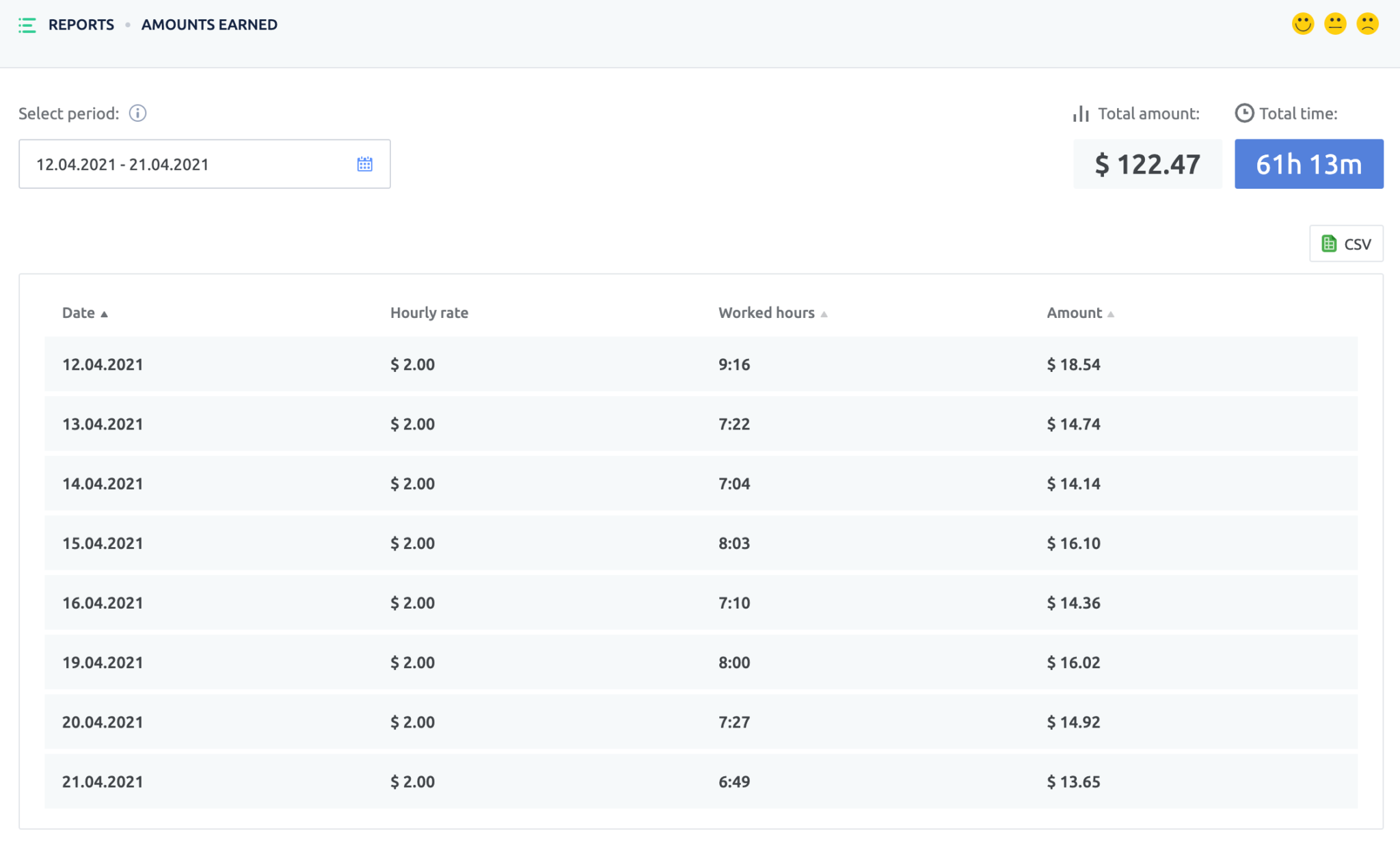The image displays a detailed business report interface. At the top left, there are three green lines, presumably serving as a menu icon. Next to it, the word "Reports" is prominently displayed in black font, followed by the label "Amounts Earned." On the upper right corner, the interface features three yellow emojis: a smiley face, a neutral face, and a sad face.

Below the emojis, in gray text with black letters, it instructs to "Select Period." Accompanying this is a search bar where users can select specific calendar dates. The currently selected period is from 12.04.2021 to 21.04.2021.

To the right of the date selection, there are two key metrics displayed: "Total Amount: $122.47" and "Total Time: 61 hours 13 minutes."

Below this header section, there is a list of dates paired with consistent hourly rates. Each date from 12.04.2021 to 21.04.2021 is recorded with an hourly rate of $2. The specific dates listed are 12.04.2021, 13.04.2021, 14.04.2021, 15.04.2021, 16.04.2021, 19.04.2021, 20.04.2021, and 21.04.2021.